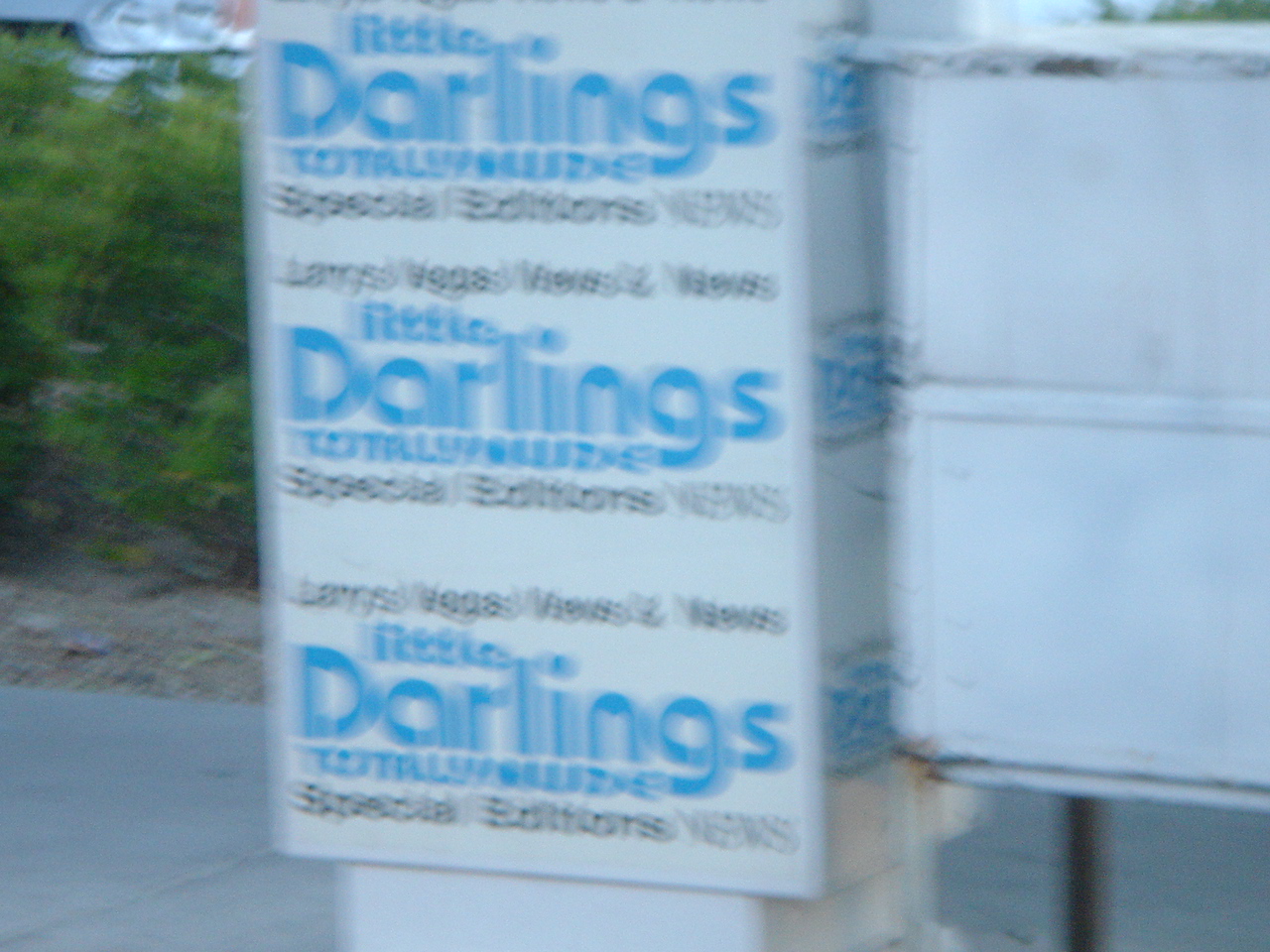The photograph is an outdoor color image, albeit very blurry and out of focus. Centrally dominating the picture is a large white box, potentially a sign or container, with multiple lines of text in blue, black, and possibly turquoise. The text, though mostly indistinct, includes phrases such as "little darlings" and might have other words like "total kite" or "special edition," though these are hard to discern due to the blurriness. This sequence of text appears to repeat three times vertically. On the right side of the image, there's another white container, suggested to have undivided compartments and lacking any text. To the left of the main white box, verdant green plants or bushes are visible, contributing a splash of color to the scene. The bottom part of the image is framed by gray roads both on the right and left, with a sidewalk and further greenery hinting at an outdoor setting near possibly urban infrastructure.